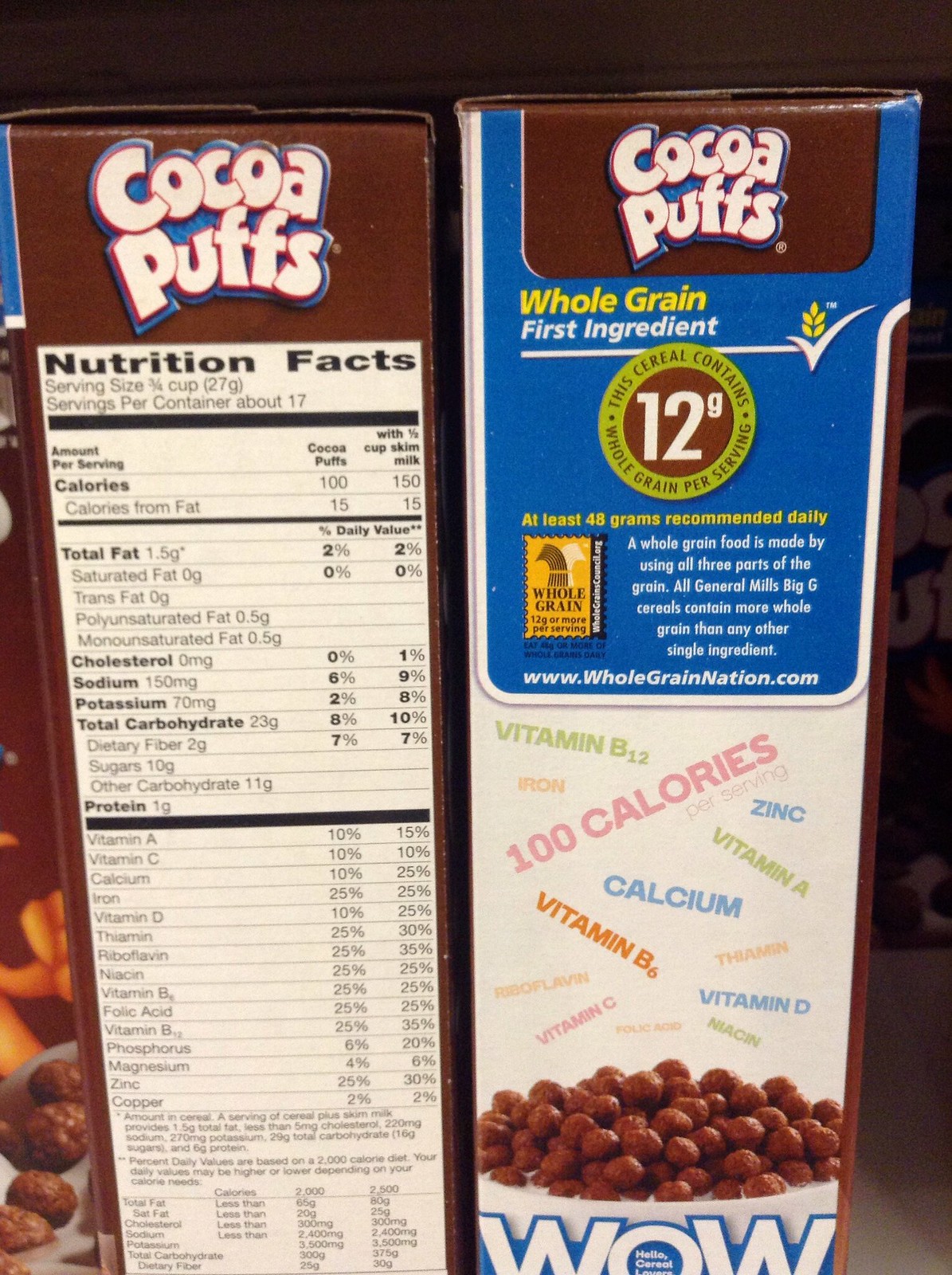The image displays two sides of a box of Cocoa Puffs cereal against a dark background. The left side of the box prominently features the Nutritional Facts panel, indicating a serving size of 3/4 cup, with approximately 17 servings per container. It includes detailed nutritional information, showing 100 calories per serving or 150 calories when combined with a half cup of skim milk, as well as data on total fat, cholesterol, and various vitamins.

The right side of the box highlights the cereal's key ingredient, stating "Whole grain first ingredient" with 12 grams of whole grain per serving. It also emphasizes that whole grain foods are made using all three parts of the grain and mentions that General Mills Big G cereals contain more whole grain than any other single ingredient. The bottom right section acts as an advertisement, showcasing benefits like vitamins B3 and calcium. Both sides of the box are adorned with the Cocoa Puffs branding, featuring the familiar brown packaging and a white bowl filled with the chocolate-flavored cereal pieces.